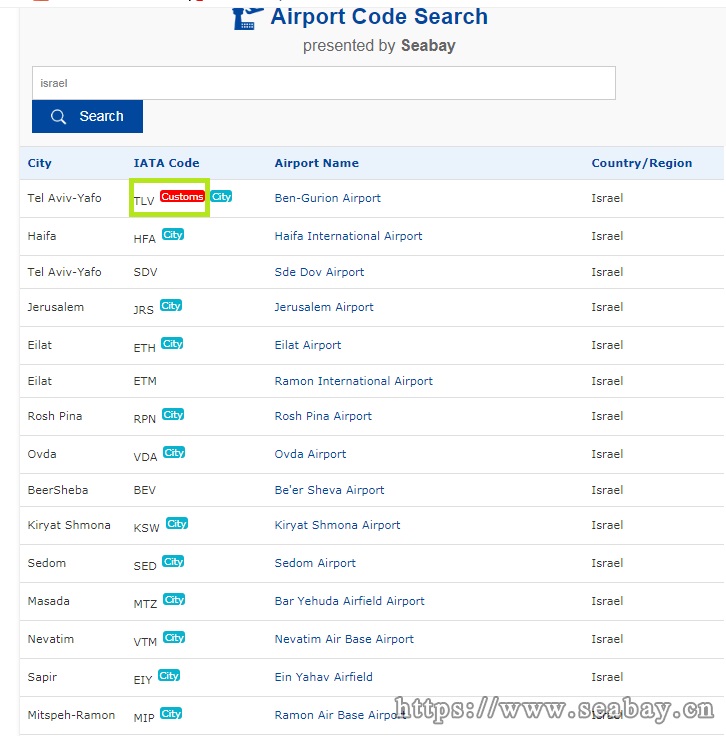Image Caption: The image features a white background with a gray rectangle containing the header "Airport Code Search Presented by Seabay," where "Seabay" is in bold blue text. Below this header, there is a search box pre-filled with the text "Israel." Adjacent to the search box is a blue rectangle with a white magnifying glass icon and the word "Search." The image lists details under various headers: "City," "IATA Code," "Airport Name," and "Country/Region."

The first entry is for Tel Aviv, with the code "TLV" enclosed within a green rectangle. An adjacent red oval within the rectangle bears the word "Customs" in white text. A blue oval with the word "City" in white is present near this entry, specifying Tel Aviv. The airport name listed is "Ben-Gurion Airport," with each letter of "G-U-R-I-O-N" underlined for emphasis. The country/region is noted as Israel.

The second entry is for Haifa, with the code "HFA" enclosed within a blue rectangle labeled "City." This section details "Haifa International Airport," also under the country/region of Israel. Another mention of Tel Aviv UFO appears as SDV in this structured format.